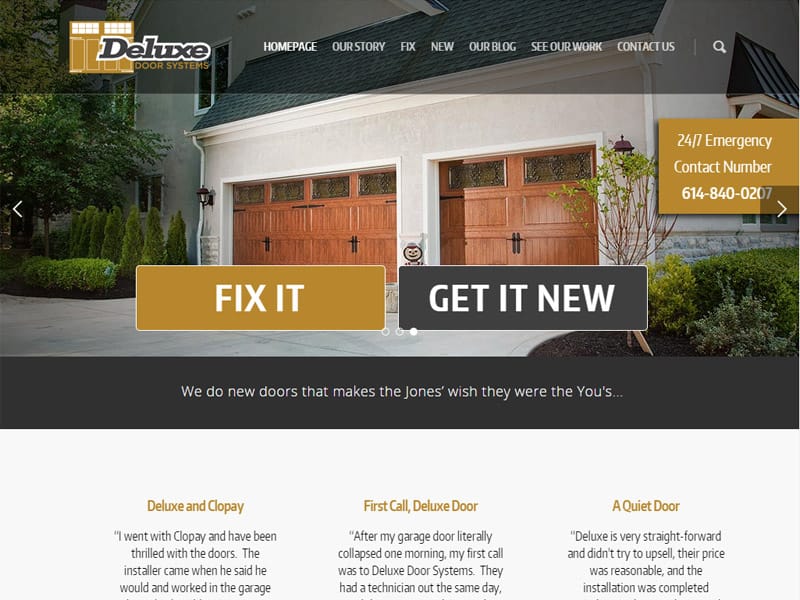**Screenshot Description: A Detailed Overview of a Garage Door Website Homepage**

The screenshot showcases a section of a website dedicated to garage doors. Dominating the page are two prominent wooden garage doors, painted in a rich brown hue, each featuring black decorative handles and windows along the top pane. The garage doors are set into a beige stucco home, complemented by lush green trees that frame the scene. The home also has a grey driveway leading up from the garage doors and a bluish roof contrasting the beige walls.

At the top of the screenshot, there's a logo accompanied by the text "Garage Doors" and "Develops Door Systems," signaling the website's focus. The navigation bar beneath the logo includes white text links for "Home," "Our Story," "Fix," "New," "Our Blog," "See Our Work," and "Contact Us." 

Adjacent to the garage doors photo, a brown box prominently displays a 24/7 emergency contact number: 614-840-0207. Below this, another brown box centered on the page contains the phrase "Fix It," while a black box underneath reads "Get It There." Lastly, there’s a message reminding users to accept the terms of use, also situated in a black box at the bottom.